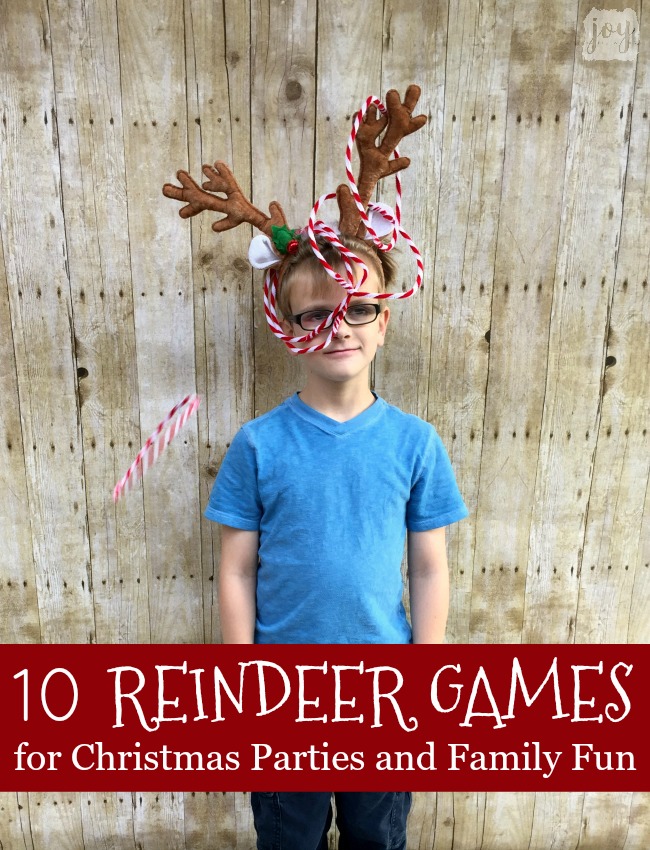The image captures a comedic and festive moment featuring a young boy, standing against a wooden fence, dressed in a plain blue t-shirt and blue jeans, and wearing black-rimmed glasses. He sports a headband with reindeer antlers adorned in a whimsical fashion with candy cane-striped rings. The boy, smiling and poised with his arms down by his sides, appears to be participating in a holiday-themed hoop toss game where red and white rings, aiming to land on his antlers, add to the playful chaos. One hoop is caught mid-air, emphasizing the action. Overlaying the lower part of the photograph is a red banner with the text: "10 Reindeer Games for Christmas Parties and Family Fun." The watermark "Joy" can be seen in the upper right corner, hinting at the image's festive origin. The setting, although vertical, is likely outdoors, accentuated by the wooden fence background.